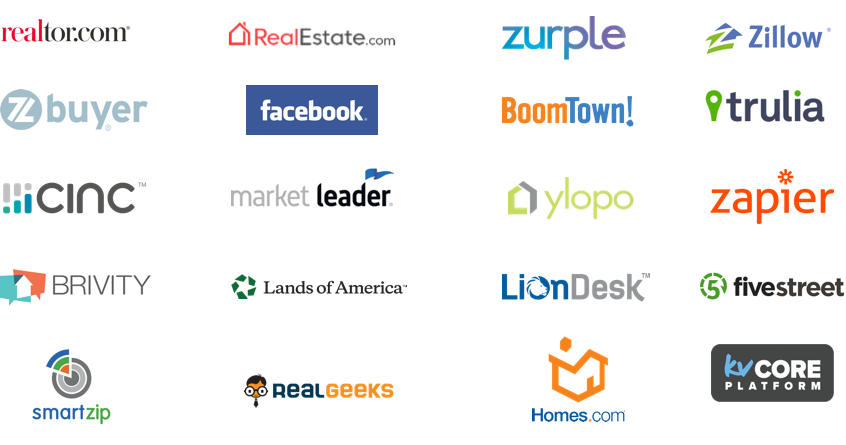This image displays a comprehensive screenshot showcasing various websites and apps dedicated to housing services, encompassing buying, selling, and renting properties. The following platforms are featured: Realtor.com, RealEstate.com, Zirple, Zillow, Zbuyer, Facebook, Boomtown, Trulia, Sync, Market Leader, Yellopo, Zapier, Brivity, Lands of America, LionDesk, 5street, SmartZip, RealGeeks, Homes.com, and KVCorePlatform.

The Realtor.com logo features "real" in red lowercase letters, followed by "Tor.com" in black lowercase letters. RealEstate.com's logo is also primarily red, with the word "real" accompanied by a small house icon, while "Estate.com" is in black. Both "R" in "real" and "E" in "estate" are capitalized. Zirple has a gradient logo that transitions from blue to purple, and the name is rendered in lowercase letters.

This detailed representation highlights the distinctive branding and visual identities of these housing platforms, aiding users in recognizing and selecting the appropriate service for their property needs.